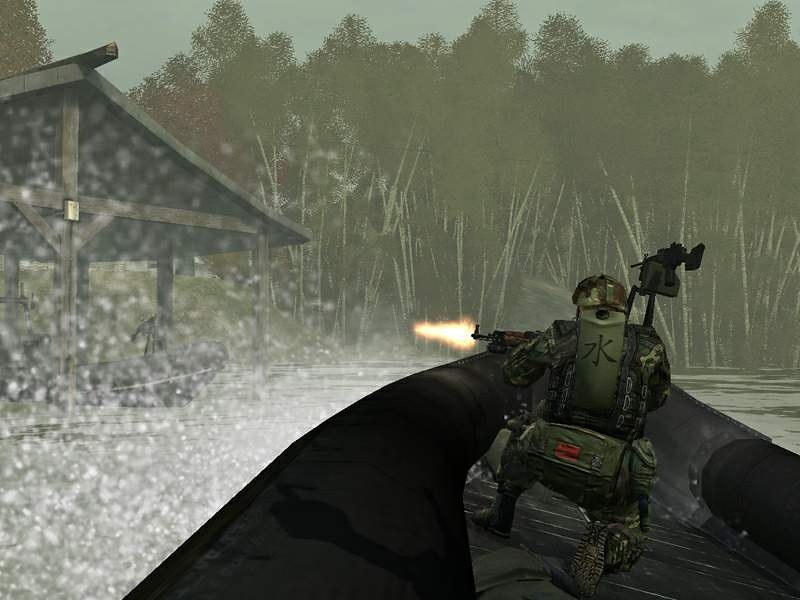The image appears to be a screenshot from a first-person shooter video game. The perspective is from a first-person view, situating the observer behind a character clad in camouflage gear. The character ahead, identifiable by a kanji character on their back, is actively engaged in shooting, with visible muzzle flash emanating from their firearm. They are targeting a wooden building situated to the left side of the scene. Both characters are aboard a small black flotation device, navigating through water that splashes visibly on the left side. The setting is a swampy, marsh-like area with tall grasses and large trees in the background. The sky overhead is gray and overcast, casting a subdued light over the scene and contributing to a moody atmosphere.